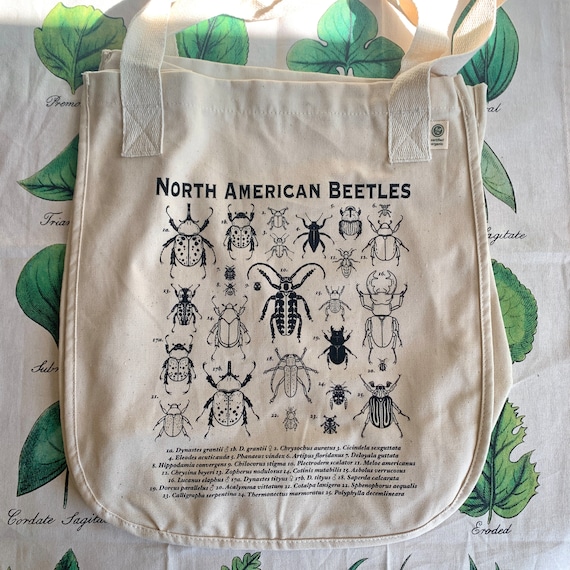This is a square-shaped, realistic-looking photograph featuring a tan canvas bag laid flat against a background that appears to be poorly lit, light-colored cloth decorated with various green leaf drawings. The cloth backdrop includes some discernible text, like "eroded," but overall, the leaf types are indistinct due to the lighting. The focal point is the canvas bag, resembling a durable, reusable satchel, which has two handles at the top. The bag prominently displays the text "NORTH AMERICAN BEETLES" in black, capital letters. Centered on the bag are approximately 20-25 black ink illustrations of different beetles, each marked with a number. These numbers correlate with their corresponding scientific names listed at the bottom of the bag, although the text is too small to be legible. The beetle illustrations appear akin to textbook-style drawings, offering accurate yet stylized representations. The photograph seems to resemble an Etsy-style advertisement showcasing the design and functionality of this unique canvas bag.